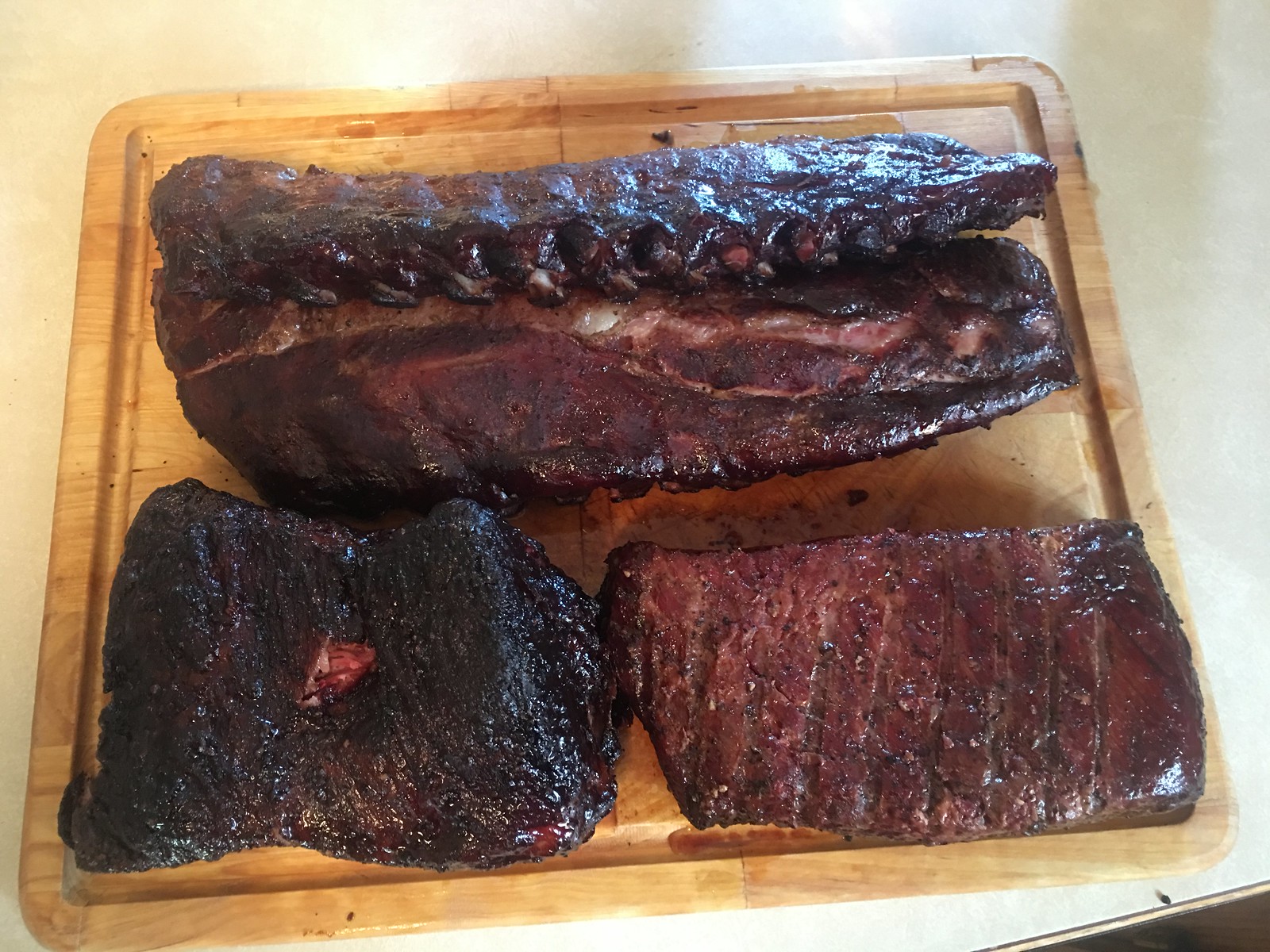This color photograph captures a square wooden cutting board placed on a light, cream-colored surface. The cutting board hosts three distinct pieces of meat, which appear to be deeply barbecued to the point of charring. The largest piece at the top stretches across the full width of the tray, potentially a rack of ribs due to the presence of bones. This piece is predominantly blackened with occasional brown patches and features a particularly charred ridge layer catching the light, alongside a noticeable white spot. Below the ribs, two smaller nearly square pieces of meat rest side by side: the left piece is almost entirely black with a small red spot at its center, while the right piece, marked by grill lines, is largely brown with scattered blackened areas, suggesting it’s less burnt compared to the others. The scene is subtly bathed in sunlight, casting varying hues and revealing underlying flooring, particularly dark in one corner.